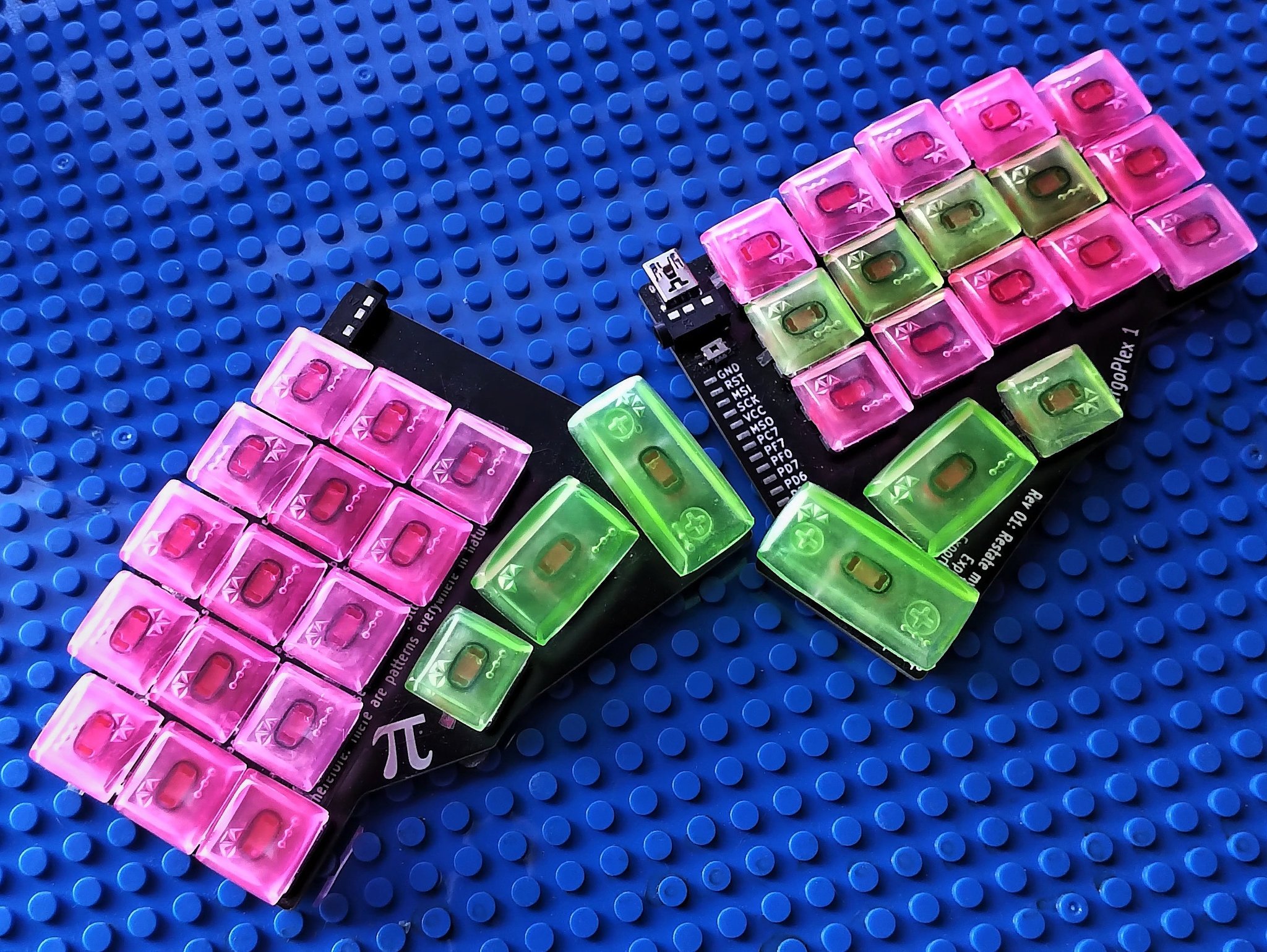The image is a multi-colored, full-color square photograph with no border. The background is a large blue Lego baseboard covered in tiny raised dots characteristic of Lego material. The main focus of the photo is several pink and green plastic tiles, reminiscent of small blocks or cubes, spread across the surface. Most of these tiles are pink and square in shape, about the size of ice cubes, while a few larger green ones are rectangular in shape. These tiles have a red piece in the middle, suggesting they might contain a component like a light.

Sitting on the blue Lego baseboard are two black pieces or bases. The black piece on the left side features the mathematical symbol for pi in white. The one on the upper right corner has a list of letter combinations formatted as three-letter acronyms or abbreviations, although their meanings are unclear. Both black bases hold a mix of the pink and green tiles, making the overall display visually striking with the contrast of colors and shapes.